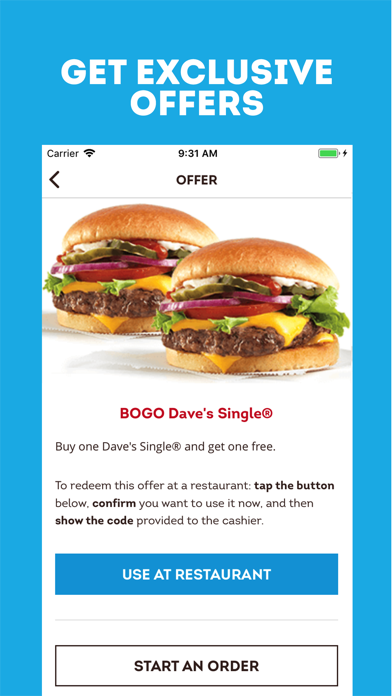This image is an advertisement screenshot for the Wendy's restaurant mobile app, designed to illustrate the benefits of downloading the app. The background is a vibrant blue. Dominating the top center, large white text proclaims, "GET EXCLUSIVE OFFERS." Below this, a mobile screenshot showcases an offer page within the Wendy's app.

At the top of this screenshot, the word "Offer" is prominently displayed. The image features two mouth-watering hamburgers with the offer title "BOGO Dave's Single" in bold red font beneath them. The offer details are clearly spelled out: "Buy one Dave's Single and get one free." Further instructions guide users on redeeming this offer at a restaurant: "Tap the button below, confirm you want to use it now, and then show the code provided to the cashier."

Two interactive buttons are shown below the instructions: "Use at Restaurant" and "Start an Order," enhancing the user experience by offering easy access to the promotion.

In the top left corner of the screenshot, "Carrier" is displayed next to a Wi-Fi icon, signifying a generic cellular provider, which underscores that this is an advertisement specifically for the Wendy's app, avoiding any promotion of external brands. The image effectively conveys the value of the app, highlighting enticing deals like a buy-one-get-one-free hamburger.